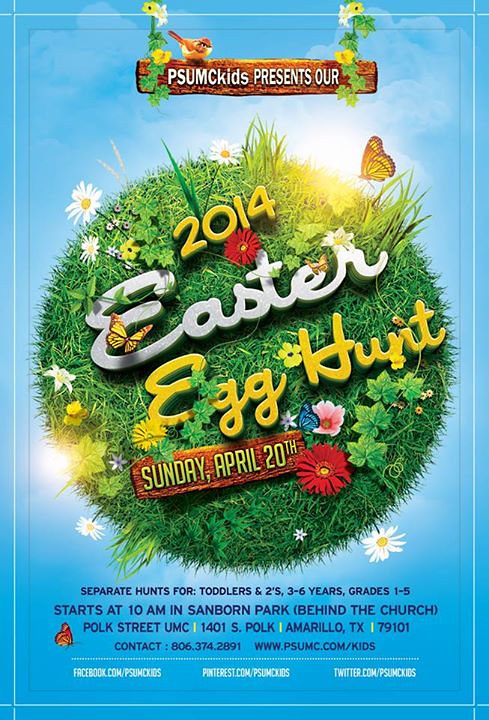This vibrant and professionally designed poster announces the 2014 Easter Egg Hunt, organized by PSUMC Kids on Sunday, April 20th. The background is predominantly blue with white accents, mimicking a sky with clouds. At the very top, a wooden sign, appearing as if hanging between two flowers and resembling a tree swing, displays "PSUMC Kids Presents Our." Below this is a circular graphic of grass and flowers, seemingly designed to look like a planet. Embedded within this circle are colorful butterflies and birds, along with the event details in alternating yellow and white text: "2014 Easter Egg Hunt, April 20th, Sunday." Additionally, the poster specifies different egg hunts for various age groups: toddlers and twos, three to six-year-olds, and grades one to five. The event begins at 10 a.m. at Sandboard Park, which is located near Polk Street United Methodist Church (PSUMC) at 1401 South Polk, Amarillo, Texas 79101. For more information, the contact number is 806-374-2091, and the website is www.psumc.com/kids.